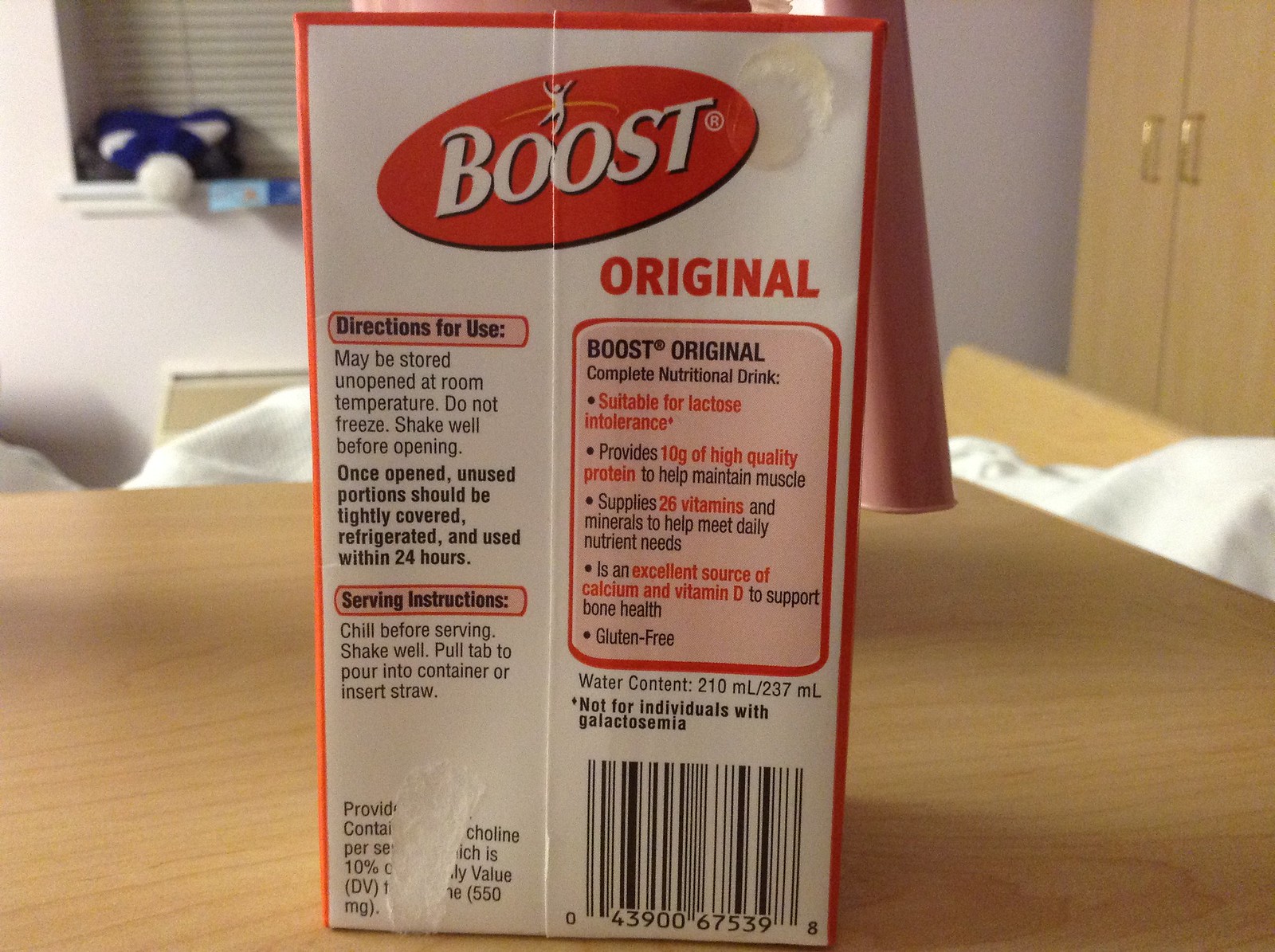This photograph captures the back of a Boost nutritional drink carton. At the top, the brand name "Boost" is prominently displayed in bold white letters set within a red oval. Above the two O's in "Boost," there's an illustration of a human figure appearing to dance, with a pink curved line arcing behind it.

The carton has a vertical seam running down its middle, dividing the information into two sections. 

On the left-hand side, the following directions are provided: 
- "May be stored unopened at room temperature. Do not freeze. Shake well before opening. Once opened, unused portions should be tightly covered, refrigerated, and used within 24 hours. Serving instructions: Chill before serving, shake well, pour tab to pour into container or insert straw."
Below these instructions, some additional information is obscured due to a tear in the label.

On the right-hand side, the word "Original" stands out in large, bold red letters, followed by the detailed benefits of the Boost Original Complete Nutritional Drink:
- "Suitable for lactose intolerance."
- "Provides 10 grams of high-quality protein to help maintain muscle."
- "Supplies 26 vitamins and minerals to help meet daily nutrient needs."
- "An excellent source of calcium and vitamin D to support bone health."
- "Gluten-free."
- "Water content: 210 milliliters / 237 milliliters."
- "Not for individuals with galactosemia."

At the bottom of this section, a barcode is present, finalizing the array of detailed product information.